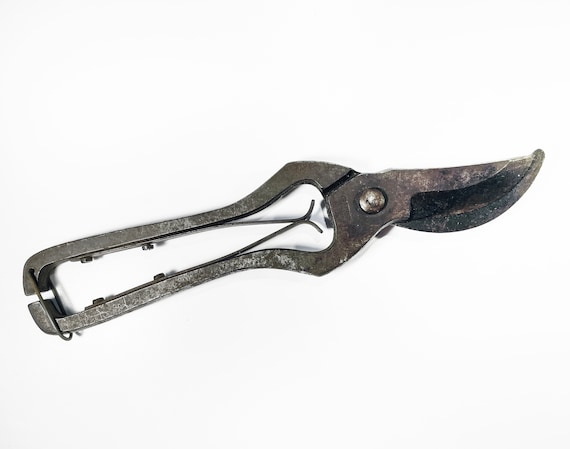The image features a pair of old, handheld shears, predominantly silver with patches of rust, indicating frequent use. The shears, about eight inches in length, have thin metal handles designed to fit comfortably in the palm of a hand. A central spring mechanism connects the two handles, with a silver clasp holding them together in the closed position. The instrument has a utilitarian appearance and is photographed against a clean, white background, emphasizing the shears as the sole focus of the image. They seem suitable for pruning small branches, approximately a quarter inch to an inch thick, and come together at the center with a singular screw. Despite their aged and slightly worn-out look, they retain a somewhat clean and mechanical appearance.